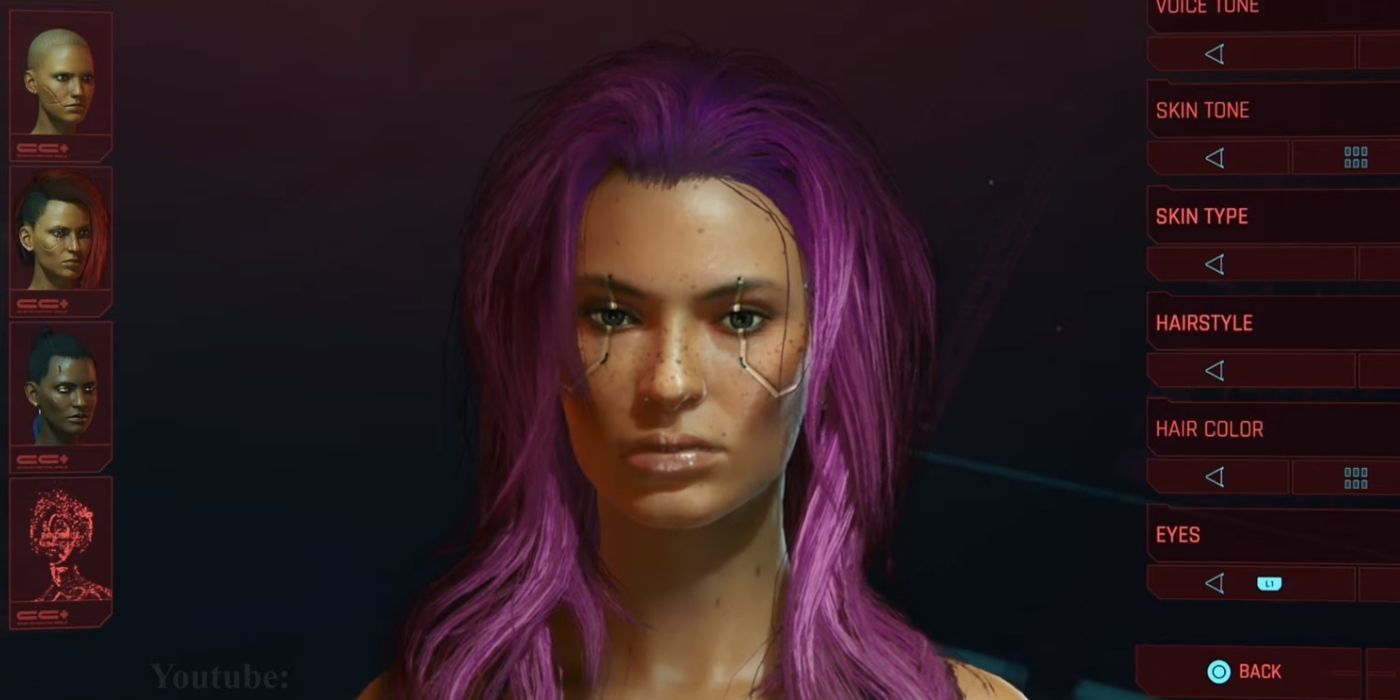This image appears to be a screenshot from a character customization screen in a video game. At the center is a woman with a beautiful yet fierce face, featuring a sad expression and long purple hair cascading over her shoulders. She has distinct scars or gold metal markings around her eyes and cheeks, suggesting implants or tattoos, and her tanned skin is dotted with freckles.

To the right of the screen, there are various customization options labeled in red text, including "skin tone," "skin type," "hairstyle," "hair color," "eyes," and "voice tone," each accompanied by a triangle for adjustment. The background is a solid black, emphasizing the character and interface elements.

On the left side, there are four images in small squares depicting different character faces: one is a black woman, another is bald, the third has dark hair with a shaved side, and the bottom image appears to be an animated or nebulous design. This setup suggests extensive customization capabilities for the game. The overall layout and design elements, such as buttons and text, indicate a user-friendly interface for creating and adjusting the character's appearance.